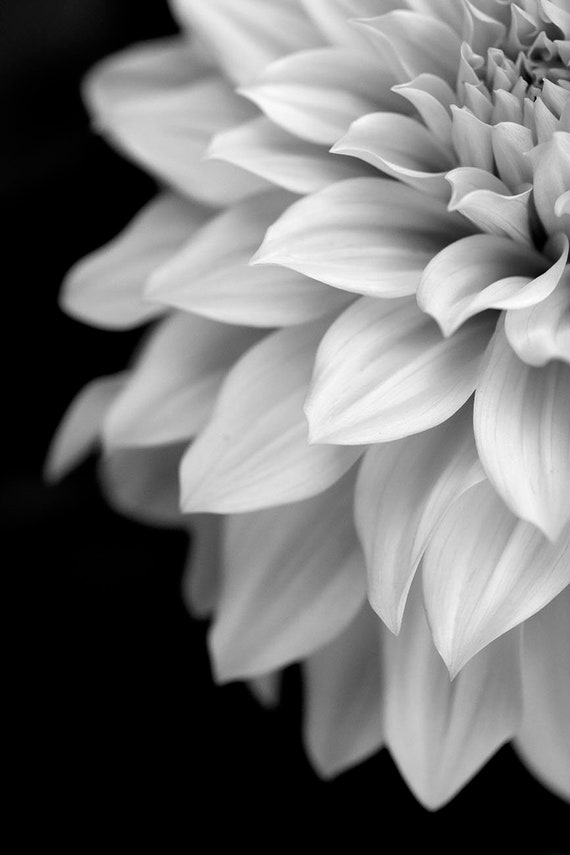This is a macro close-up shot of a white flower against a completely black background, creating a striking black-and-white photo. The flower, which is somewhat off-white with color gradients and intricate details, dominates the image, extending from the top right to near the bottom left, almost touching the edges and taking up most of the frame. The center is densely packed with small, upward-facing petals, transitioning into larger and looser petals as they radiate outwards and downwards, some remaining tightly closed while others are fully open. The petals have a teardrop shape and exhibit various intricate striations, adding depth through subtle shadows. The black background is out of focus, further emphasizing the flower's delicate and complex structure.